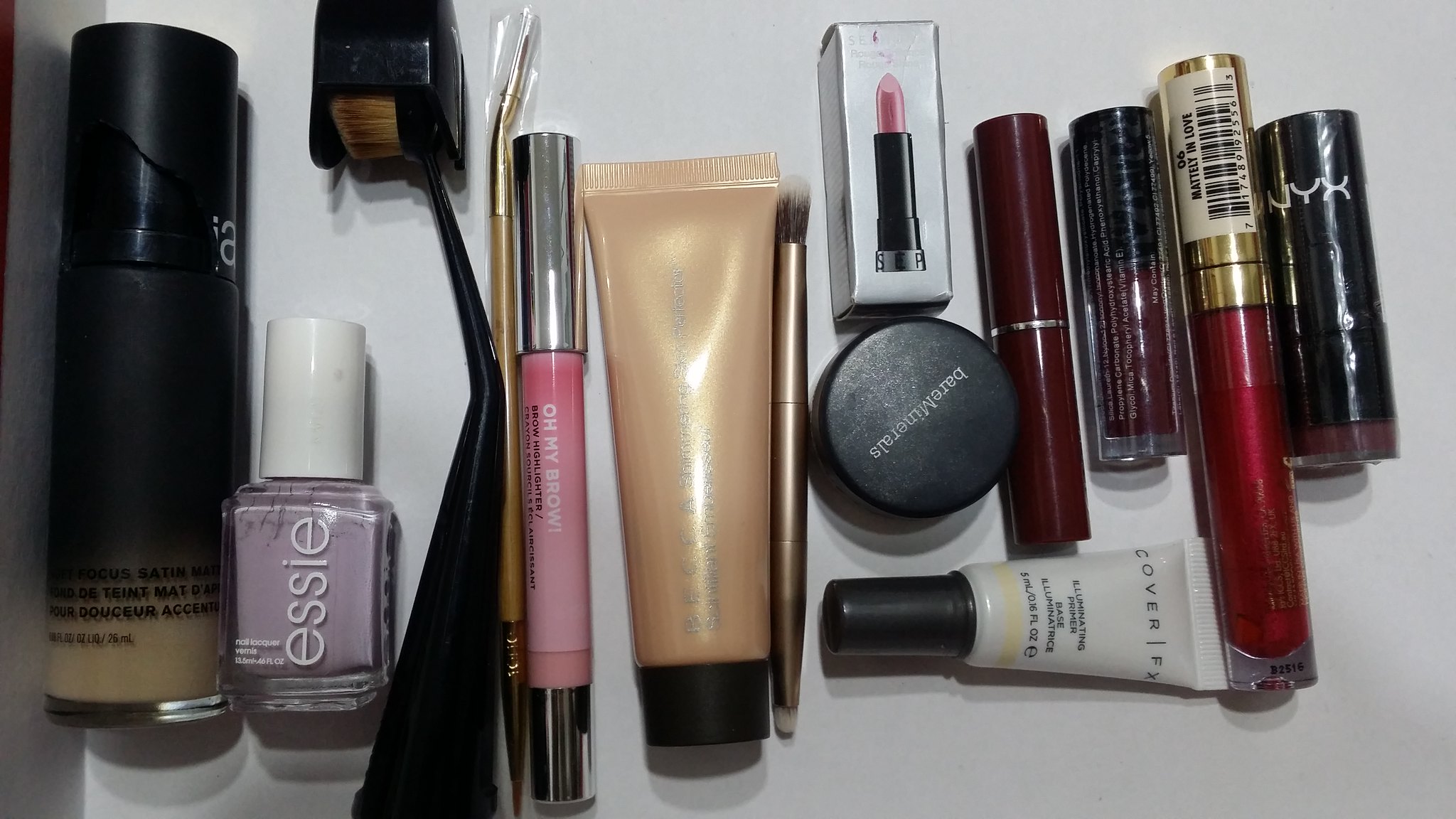This close-up shot captures an array of beauty products neatly arranged side by side on a counter, possibly inside a drawer or box, given a visible edge on the left. 

On the far left is a long, black tube with a lighter brown tip at the bottom, though its exact purpose is unclear. Adjacent to it sits an Essie nail polish in a metallic lilac shade, with the brand name prominently displayed on the bottle. 

Next to the nail polish, two makeup brushes are arranged side by side. The left brush is larger, with a black handle and a fluffy bristle head, which is protected by a cover. The adjacent brush, significantly smaller, has a lighter brown handle. 

Following the brushes is a pink tube labeled "Oh My Brow," featuring silver caps on both ends. Beside it stands a small metallic gold tube, likely containing lotion, though the text is obscured by glare. 

To the right is another double-ended brush with a gold handle, varying in bristle size at each end. Directly next to it is a tub of Bare Minerals, and above that tub lies a sample-sized pink lipstick. 

Below the Bare Minerals jar is a very small tube of Cover FX Primer. Positioned to the right are two maroon tubes of different size; one is a longer tube featuring a red bottom and a gold top, likely a lip gloss, while the other is shorter and darker. 

Finally, an NYX tube, short and black, completes the lineup; it could either be a blush or lipstick. The meticulous arrangement showcases each product distinctly, ready for use.